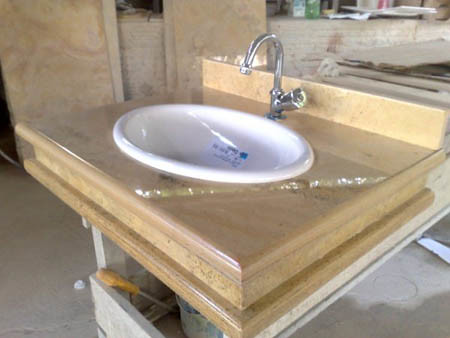The image depicts a white sink basin under construction or on display in a store setting possibly resembling a Home Depot. The basin is prominently featured with visible protective plastic wrap covering it. The sink is positioned against a white wall backdrop and set within a wooden base structure. On the ground below the sink, there is a screwdriver. In the background, a table is discernible, contributing to the context of an ongoing installation or a store display environment.